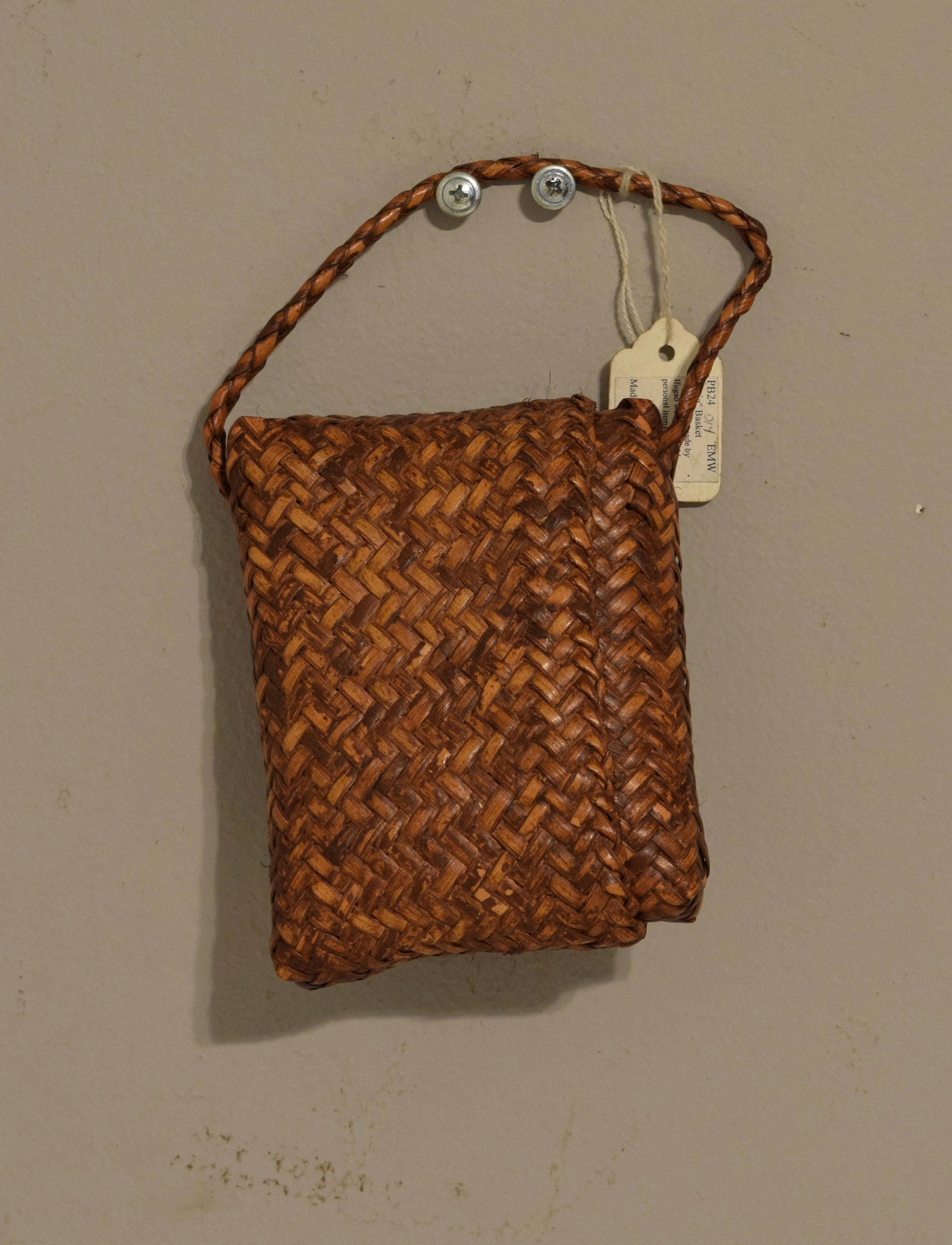The image features a detailed brown wicker purse or satchel hanging prominently on two silver-colored Phillips head screws against a plain gray wall with small brown stains near the bottom. The purse or satchel, made from a braided wicker-like material, showcases a zigzag pattern and a thin, slightly off-center strap. It displays a rectangular and vertical form and is possibly constructed from vine or basket-making materials. The light brown bag lacks visible zippers and is fitted with a tan, rectangular price tag tied around the handle with a string, displaying the letters EMW and numbers PB24.